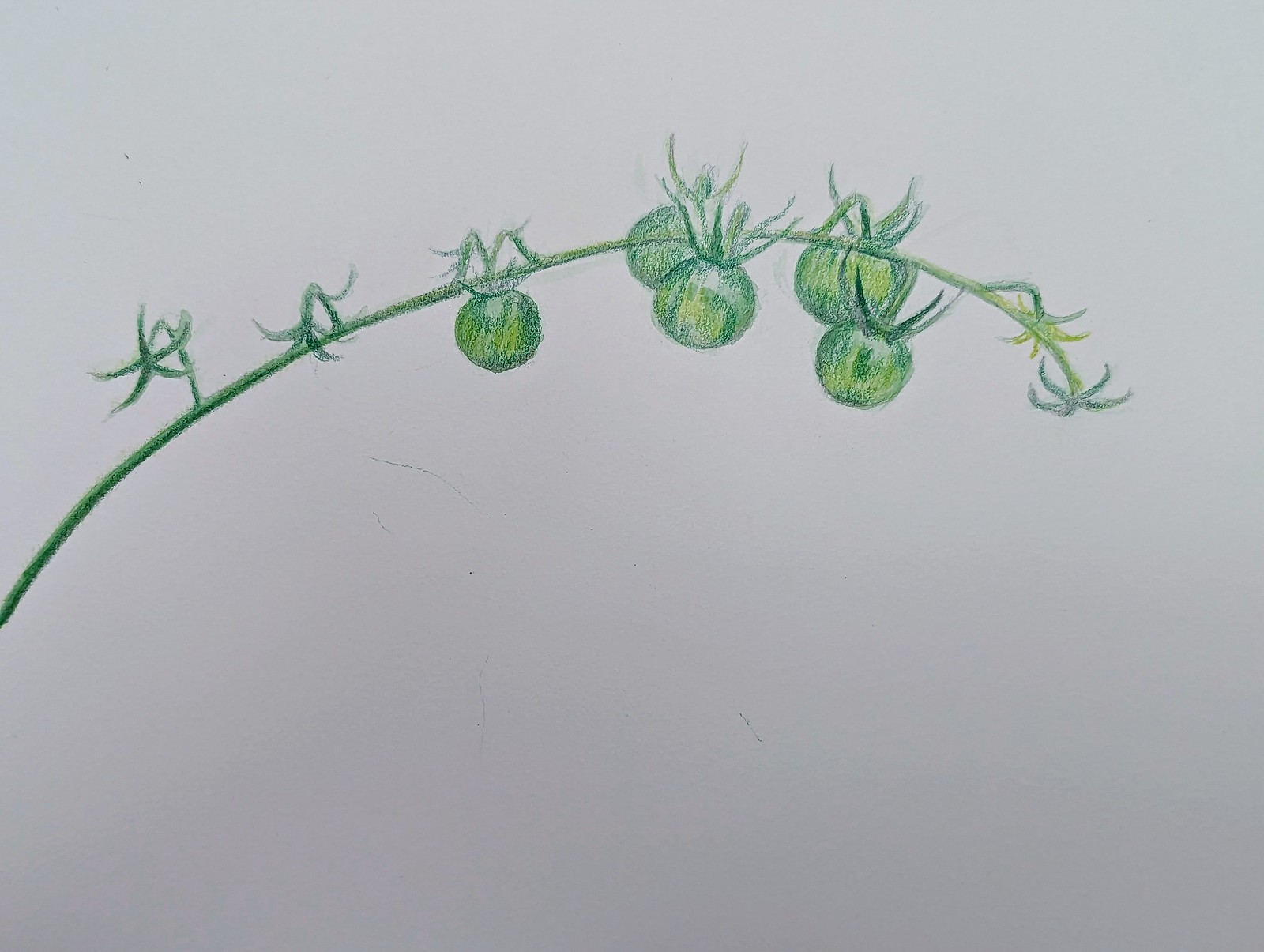This detailed colored pencil drawing portrays a cluster of cherry tomatoes on an off-white paper. The composition predominantly utilizes various shades of green to depict the slender, curling vine and its delicate stems. The focal point of the artwork features five immature cherry tomatoes, which are still green and awaiting ripening. Two additional stems, devoid of fruit, extend from the left side of the vine.

The artist has meticulously rendered the textural nuances and fine lines of the tomatoes and vine, revealing a thorough attention to detail and a keen observation of the subjects' natural forms. The absence of any text, human presence, or other objects in the image leaves the viewer to infer the scale from the familiar appearance of the cherry tomatoes themselves.